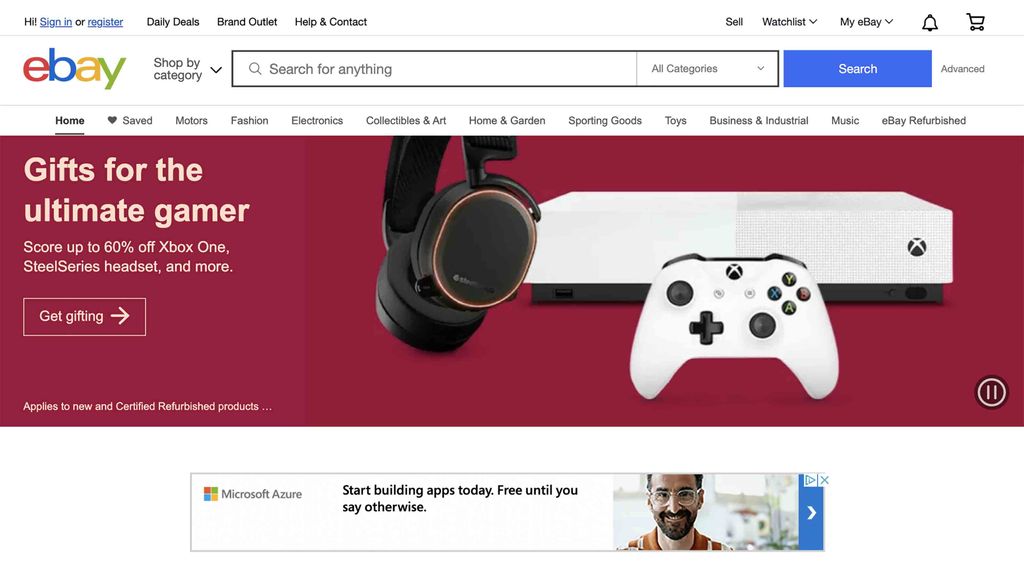The eBay webpage showcases a "Shop by Category" section with a convenient drop-down menu for quick searches, complemented by a blue "Search" button at the end of the line. Below this is a prominent red banner featuring a sleek Xbox console, predominantly white with black accents, positioned next to a pair of black headphones with distinct red rings around the ear cups, labeled as "SteelSeries". The banner reads "Gifts for the Ultimate Gamer" and offers discounts of up to 60% off on Xbox One, SteelSeries headsets, and more, with a call-to-action to "Gift Giving" indicated by an arrow. However, no price is displayed for the discounted products.